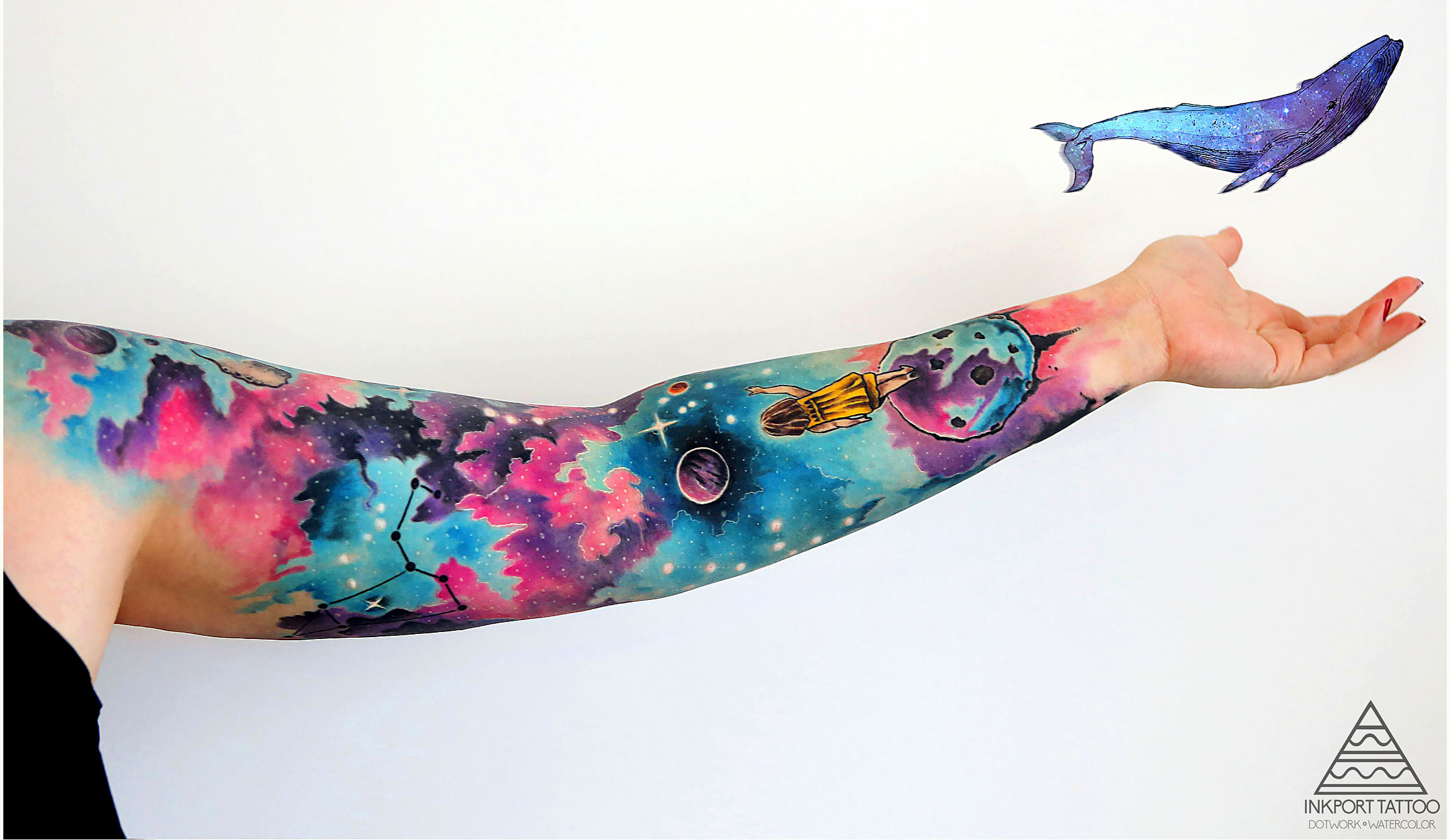The image features the extended left arm of a person, likely a white male, wearing a black tank top, with distinctive tattoos covering the shoulder down to the wrist. The arm, extended to the left with the palm open and facing upward, displays a vibrant tattoo sleeve featuring a space-themed design. The tattoo includes a mix of bright neon colors such as pink, blue, and purple, with cloud-like formations, constellations, and planets. On the inside of the lower forearm, there's a detailed depiction of a young girl in a yellow dress with brown hair, standing on a blue planet with black spots, pointing upwards as if reaching for the stars.

Hovering above the extended hand is an illustrated blue whale, floating against the white backdrop, painted with a gradient of blue and purple hues. The lower right corner of the image showcases a black pyramid logo with the inscription "Ink Port Tattoo." In smaller text beneath the logo are the words "Dot Work" and "Watercolor," accompanied by a small circle design. The photograph is set indoors, with a light gray background in the lower right-hand corner, enhancing the vivid colors of the tattoos and the overall artistic elements.